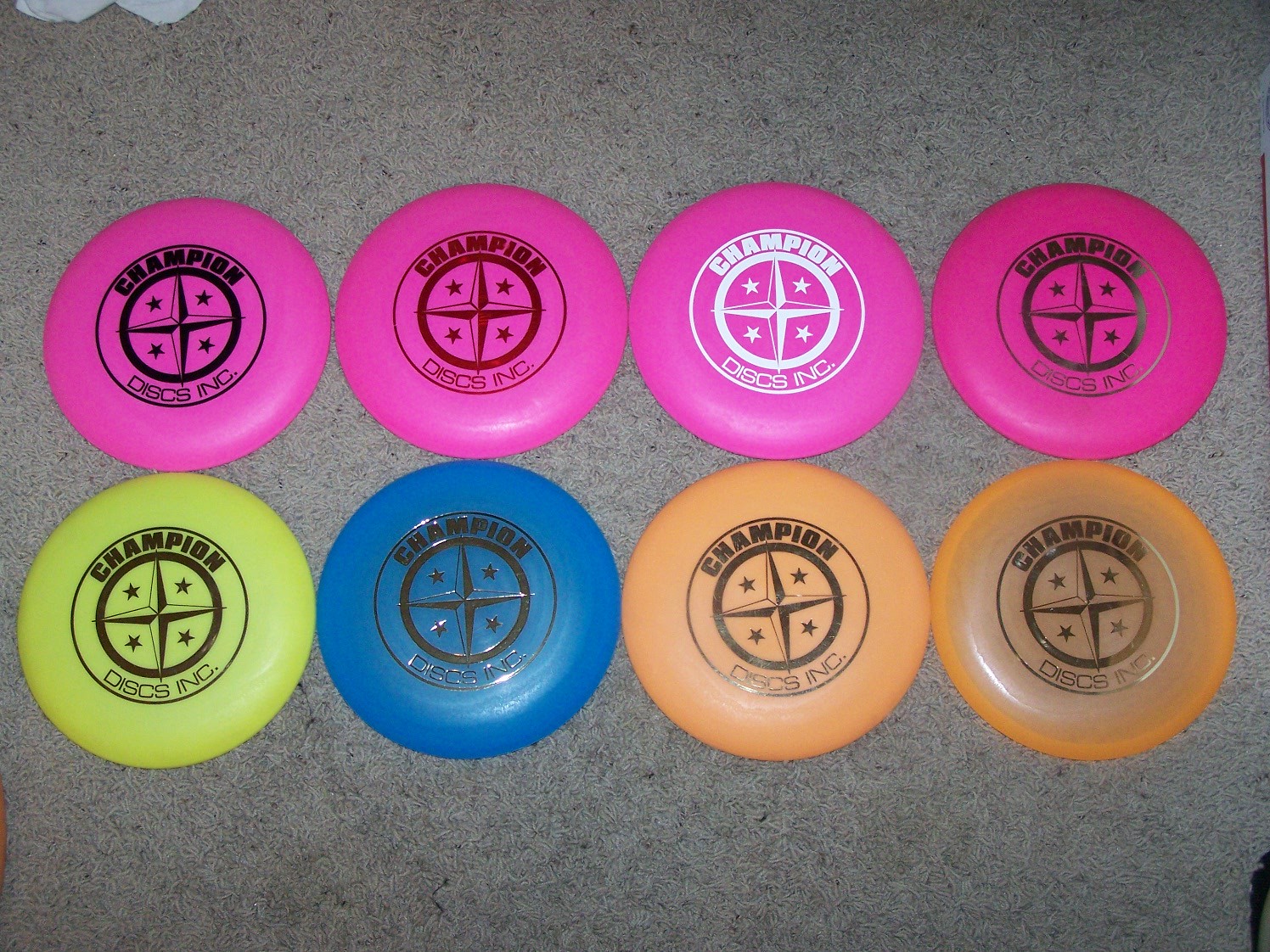This is an overhead photograph of eight colorful frisbees arranged in two rows of four on a gray, speckled stone surface. The four frisbees in the top row are all bright pink, each featuring a different colored logo of a four-point compass with stars between each point, and the text "Champion Discs, Inc." around it. From left to right, the logos on the pink frisbees are printed in black, dark red, white, and brown. The bottom row consists of a yellow frisbee with a black logo, a blue frisbee with a black logo, an opaque orange frisbee with a black logo, and a transparent orange frisbee with a black logo. The very edges of someone's toes in white socks can be seen at the top left corner of the image.